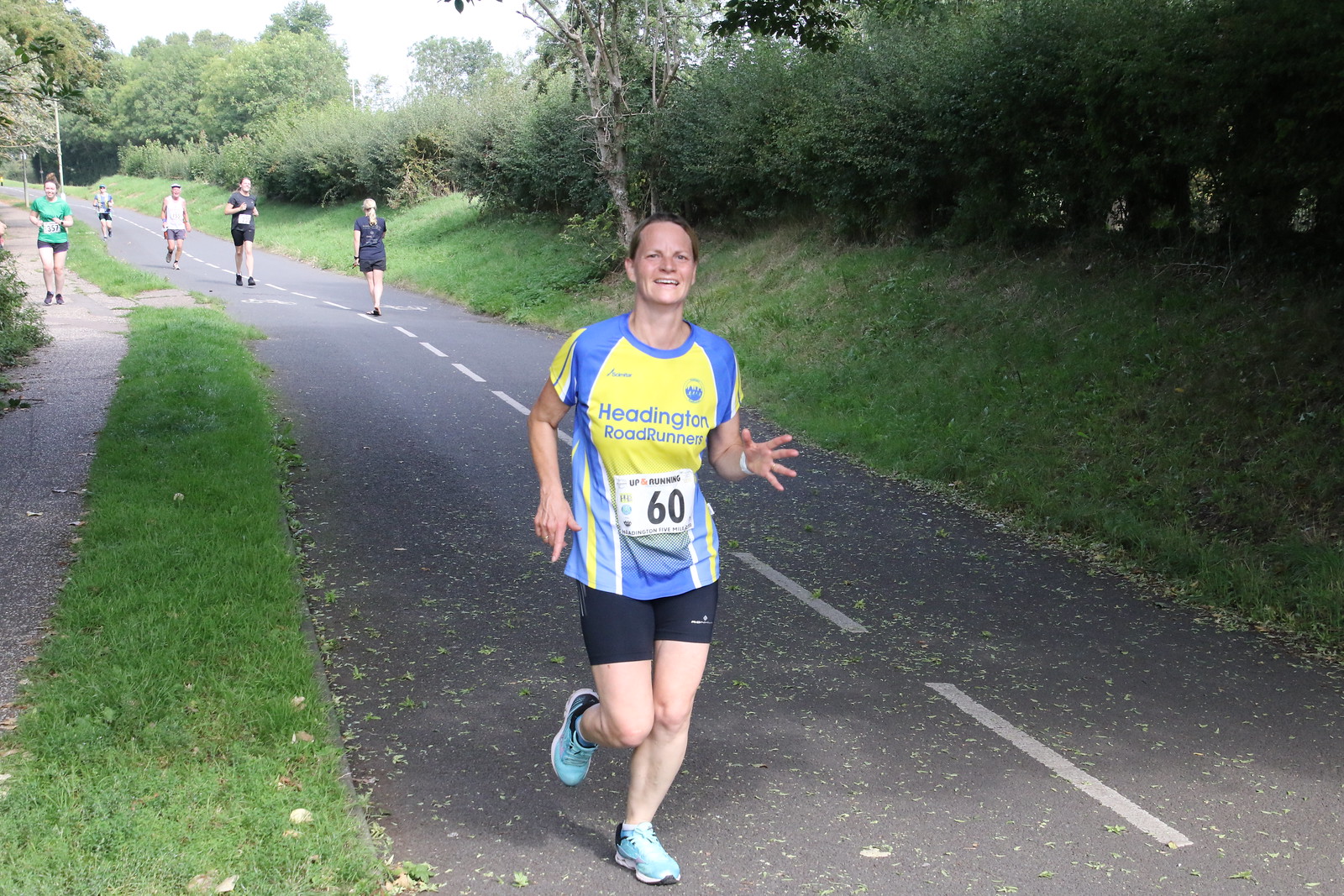In this photographic image, a group of six people are captured running along a gray asphalt road with white stripes, bordered by grass and a sidewalk median. The scene is set outdoors on an overcast daytime. Prominently in the foreground is a cheerful woman, appearing to be in her mid-40s, wearing a yellow and blue jersey that reads "Headington Road Runners" and marked with the number 60. She sports black shorts, light blue sneakers, and a wristwatch. To the right and slightly behind her is another woman in a black t-shirt and skirt, possibly a reporter, as she appears to be walking away from the race while observing others. Further back, a diverse group of runners and walkers can be seen, including a younger man dressed in black, an older man in a white tank top and gray shorts, a man in black shorts with a green jersey, and a woman on the sidewalk, wearing a green t-shirt, black pants, and black sneakers. The surroundings include trees, varying green shrubs, and a gentle slope, creating a serene background for this energetic scene.